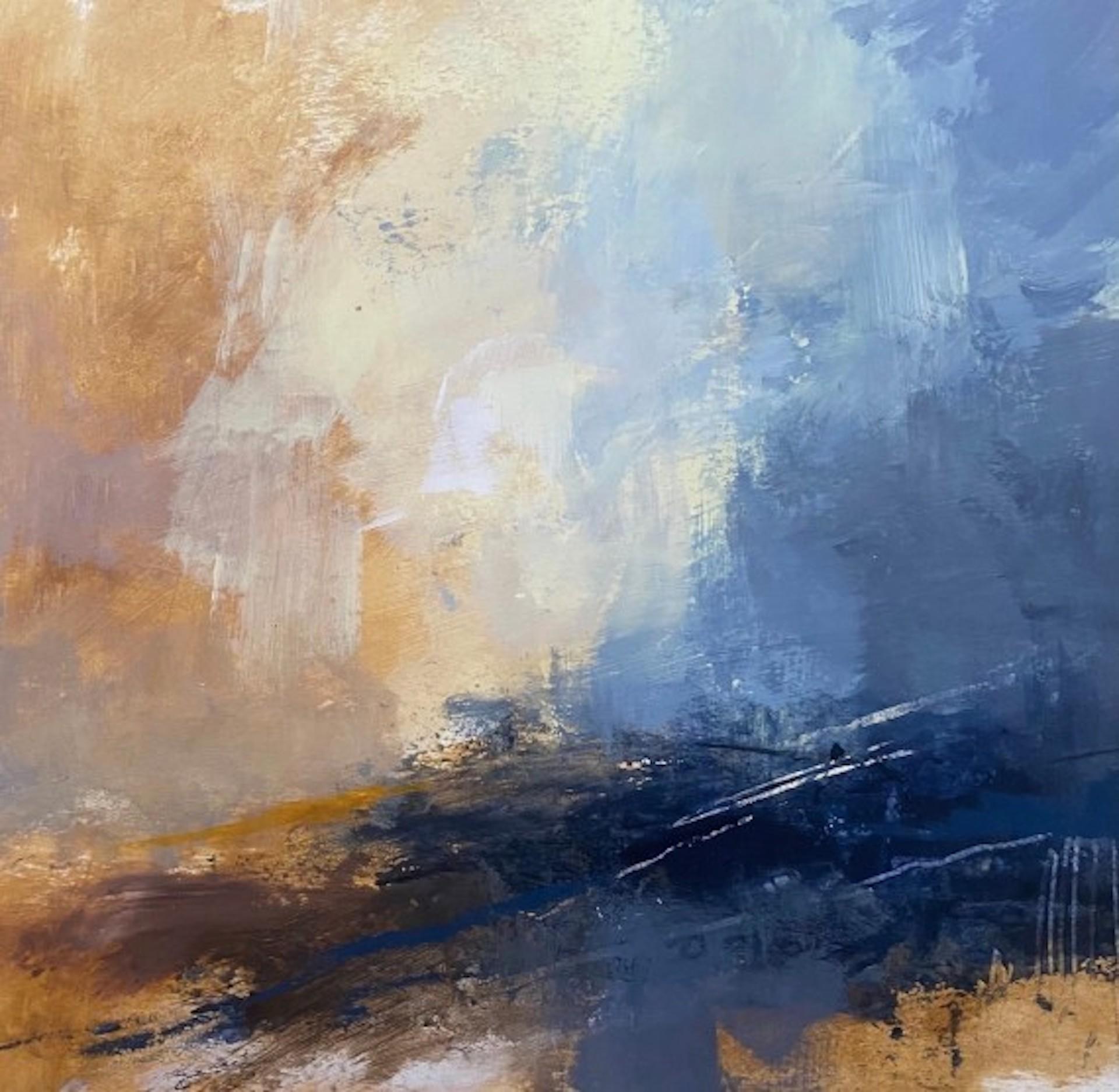This abstract oil painting is a dynamic blend of colors and textures, predominantly featuring shades of orangey-brown, white, lighter blue, and darker blue. The painting's composition transitions from darker, heavier tones at the bottom to lighter shades towards the top, suggesting a faint landscape. The left side of the canvas holds a blend of brown smeared with hues of cream and tan. The central portion is dominated by white and cream tones, featuring a pale yellow spot that could be reminiscent of the sun. To the right, the colors shift to a baby blue sky, which darkens progressively towards the bottom, mingled with gray undertones. The brushstrokes are evident, with some areas displaying a sponged texture or the effect of scraping, adding depth to the artwork. The lighter upper area transitions into what seems like an abstract sky, with the colors bleeding and merging to create a harmonious flow across the canvas. The interplay of these elements makes the painting both impressionistic and enigmatic, leaving much to the viewer's interpretation.